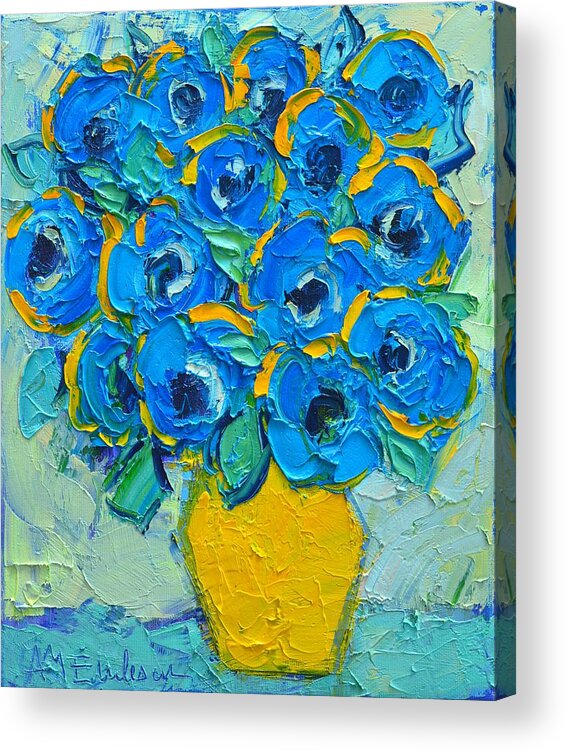The painting is a textured canvas that portrays a vibrant bouquet of blue flowers with dark centers, encompassed by golden-orange edges for added dimension. These flowers are tightly clustered in distinct tiers and layers. The foliage between the flowers ranges from bluish-green to a darker green, complementing the floral arrangement. The flowers are held in a bright yellow vase, resting on a cyan surface, accentuated by a dark blue outline at the bottom. In the lower-left corner lies the artist's obscured signature, almost hidden under thick layers of paint. The background of the painting is a blend of cyan with splotches of beige and green, transitioning to more prominent white and streaks of blue towards the top, enhancing the overall composition. Notably, the dense application of paint creates a bumpy, stucco-like texture that emphasizes the painting's depth and richness on a canvas board, with some of the painting extending to the sides, suggesting it might be a print rather than the original artwork.